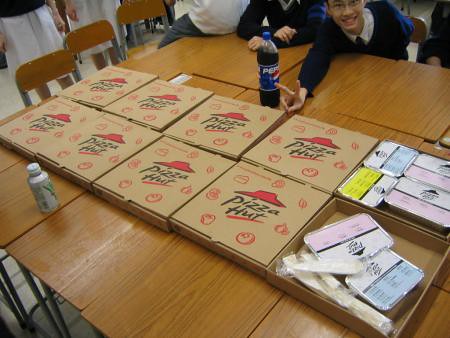This vibrant indoor photograph captures a lively school gathering. The focal point is a large wooden table, which is actually comprised of approximately 12 smaller school desks joined together. Spanning across the table are 10 Pizza Hut pizza boxes, neatly arranged in two rows. Each box is adorned with the iconic red "Hut" logo and the Pizza Hut name in black font, complemented by small red tomato illustrations. Two of the boxes are open, revealing takeaway containers, likely holding dipping sauces or chicken wings, along with wrapped napkins and plastic utensils.

Behind the pizza boxes, there's a recognizable Pepsi bottle, bearing the classic red, white, and blue logo. In the upper background of the image, a few kids can be seen, adding a touch of liveliness to the scene. One child, an Asian boy with glasses and a blue school uniform, stands out; he smiles warmly at the viewer while holding up a peace sign. To the right, another individual in a blue shirt and white skirt is partially visible. The overall setting, with its tan desks and chairs, suggests a casual, fun-filled school event centered around a delicious pizza feast.